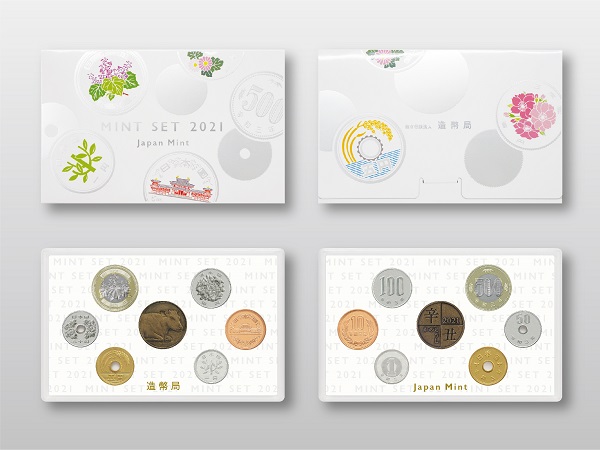This image showcases two distinct coin sets from the Japan Mint, 2021. They are displayed on a gray surface. Each set is paired with its respective cover positioned above it. 

The cover on the top left reads "Mint Set 2021 Japan Mint" in silver text and features floral designs. Below this cover is its corresponding coin set, consisting of seven coins arranged symmetrically: three coins horizontally in the middle, with additional coins positioned above and below the left and right middle coins. Notable coins in this set include a 500-yen coin and a brown coin featuring a cow or bull, along with other coins adorned with various designs such as sakura blossoms. Japanese characters decorate the bottom middle of this set.

On the right side, the cover also includes ornate floral designs and text that is somewhat difficult to discern. Below this cover lies the second coin set with an identical layout to the first, containing seven coins. Prominently featured are a silver 100-yen coin, a 50-yen coin, and a 10-yen coin. The bottom center of this set reads "Japan Mint" in gold lettering.

Each coin set displays a variety of coins, primarily in white and silver colors, emphasizing the intricate designs and craftsmanship of the Japan Mint.